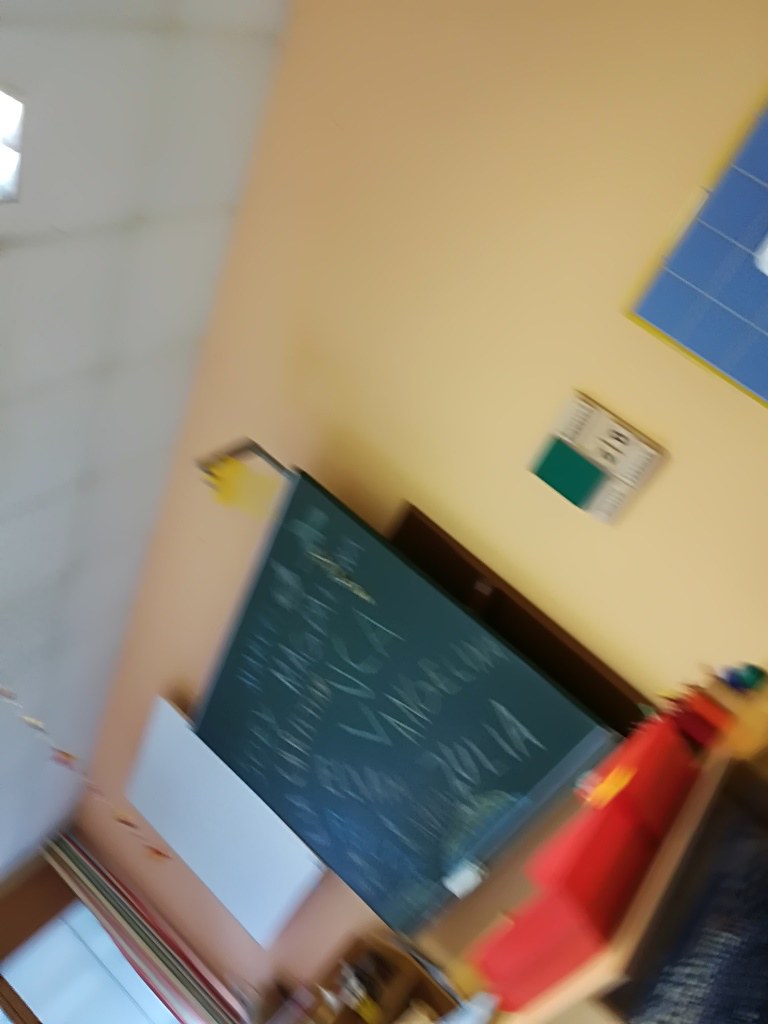This is a blurry photograph taken inside a classroom at a tilted angle, roughly 45 degrees to the left, as if the photographer leaned their head onto their left shoulder while snapping the picture. Predominantly, a green chalkboard occupies the center of the image with various words and possible names—like "Luca" and "Julia"—written in chalk. Adjacent to the chalkboard on its left side, a whiteboard is mounted on the wall. Partially visible behind the chalkboard is a door. At the bottom left corner of the image, an orange object rests on a desk. On a shelf to the right of the chalkboard, there are red containers, possibly bottles of paint. Additionally, a calendar appears to be pinned on the wall to the right of the chalkboard. The walls, painted in a light peachy-brown color, contrast with the white ceiling.